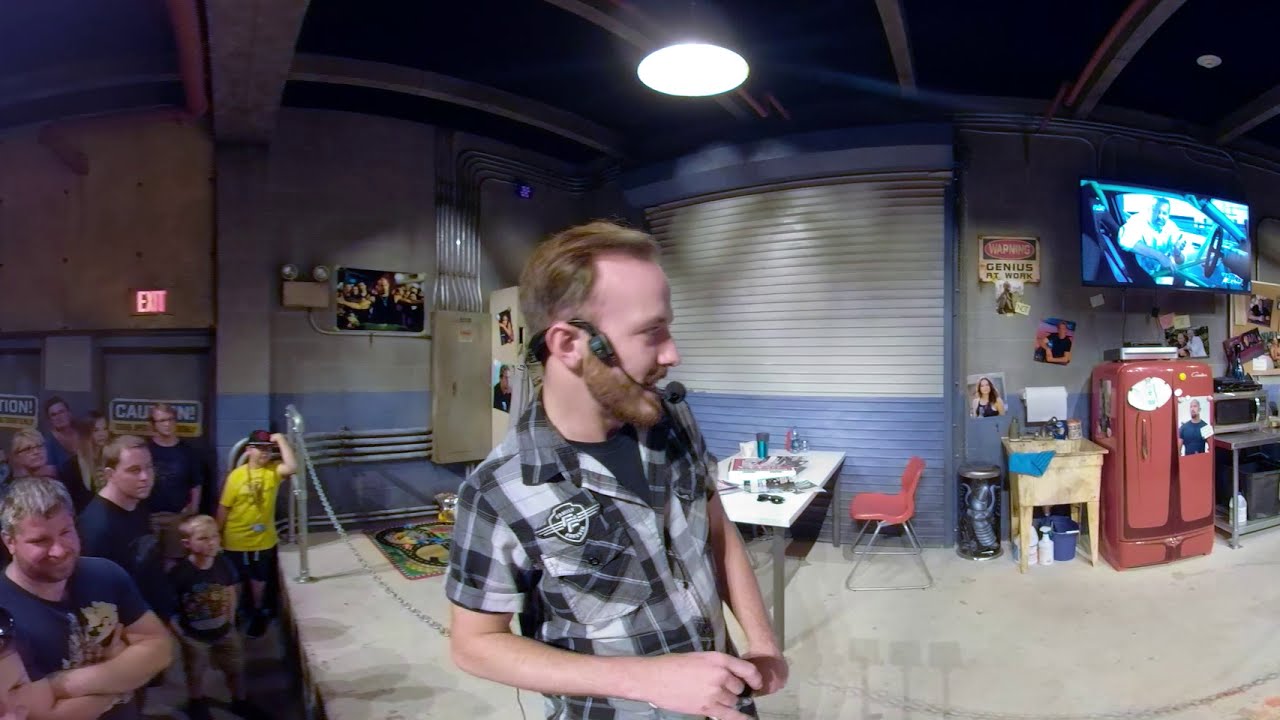In a bustling, industrial warehouse reminiscent of Tim the Toolman’s workshop from Home Improvement, a light-brown-haired, bearded man is the focal point. He's energetically narrating into a headset microphone while intensely playing video games. Dressed in a gray and white plaid short-sleeve button-down shirt layered over a dark t-shirt, he holds a controller and gazes towards the right. Around him, the warehouse features cinder block walls adorned with Fast and Furious movie pictures and a "Genius at Work" warning sign. To the right of the frame, there's an eclectic setup including a vintage red refrigerator, a white table scattered with miscellaneous items, a red chair, a steel table with a microwave, and a plastic utility sink. A large screen TV is mounted on the wall. The elevated platform he stands on is cordoned off with chrome poles and chains, separating him from an enthusiastic crowd of about eight people—children and adults alike—all smiling and enjoying the spectacle. The scene is lit by a bright light source overhead, casting a vivid glow on the man and his surroundings.